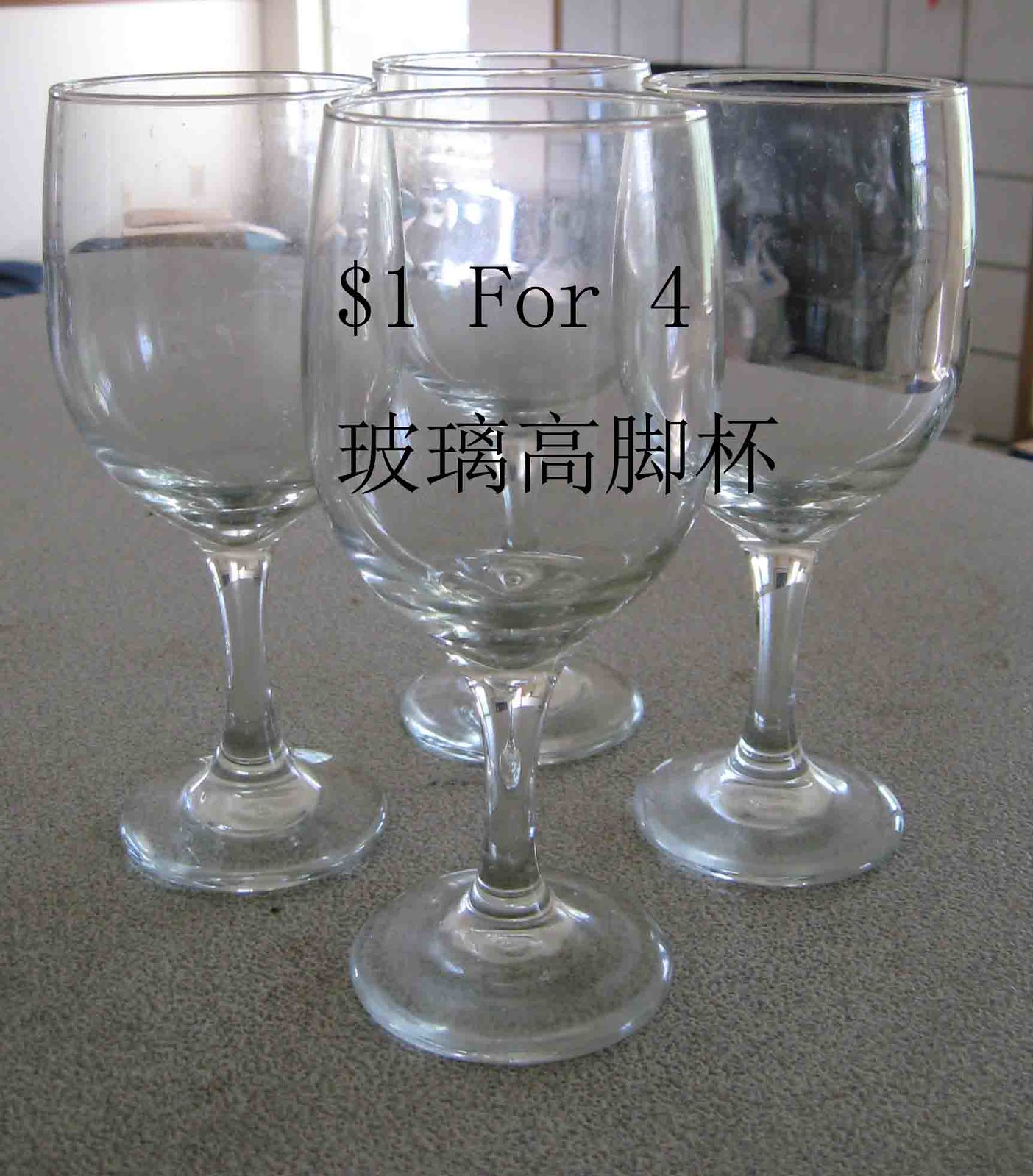This photograph captures an advertisement seemingly from a Facebook Marketplace listing, featuring four clear glass wine goblets arranged in a diamond formation atop a dirty, gray speckled countertop. The glasses, which are fairly dirty with stains, have a thick base, a reasonably thin stem, and a large upper area without curvature at the top. Superimposed on the image is black text that reads "$1 for four," followed by what appears to be Chinese characters of the same size and font. In the background, a tiled fireplace and a window with incoming light are visible. The scene emphasizes the overall untidiness of both the glasses and the countertop.